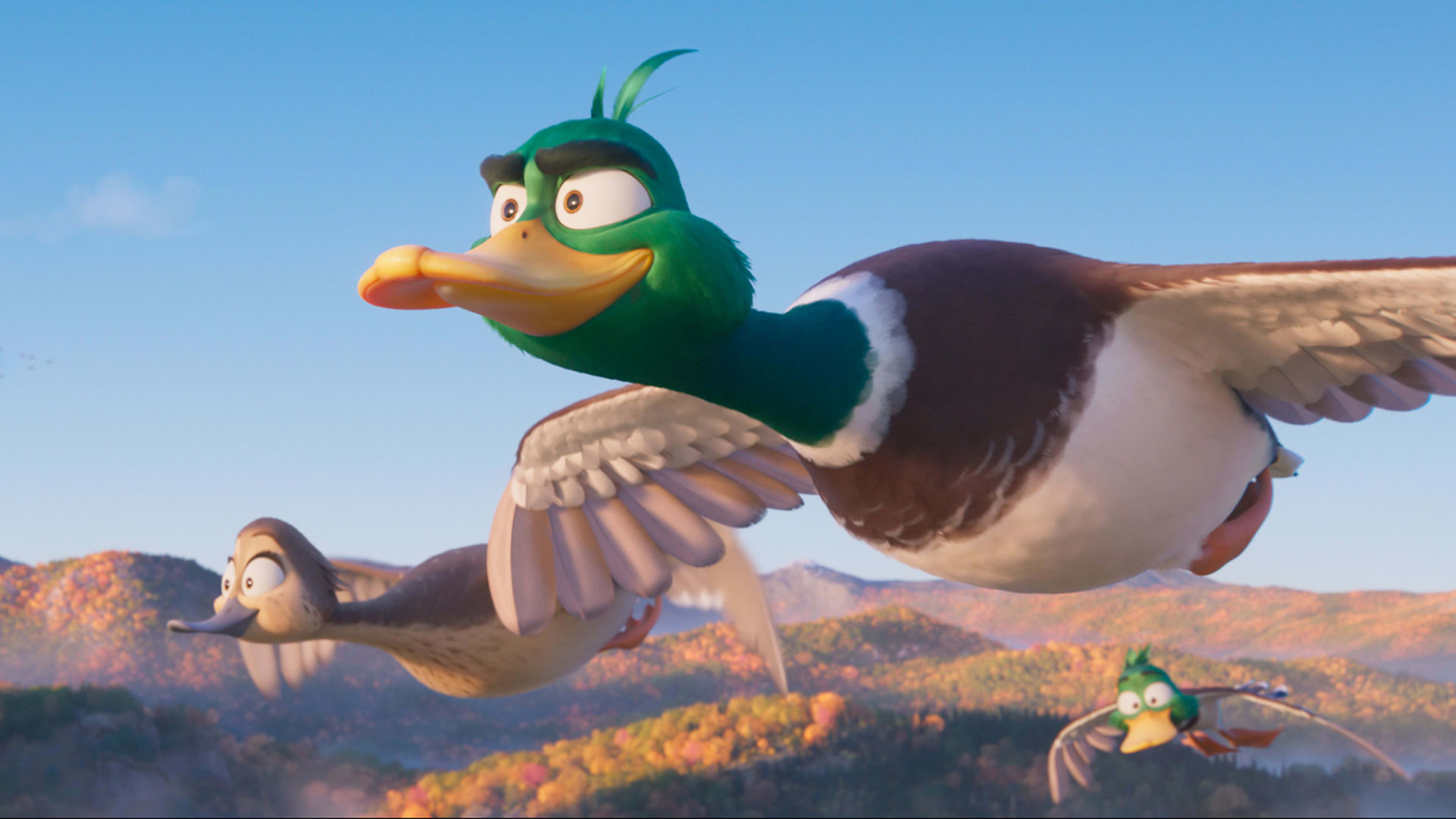This is a scene from the animated movie *Migration*, depicting a family of cartoon Mallard Ducks flying through a clear blue sky. The image prominently features the father, characterized by his green head, long orange beak, broad black eyebrows, and dark brown upper body with a light beige underside. His wings are outstretched as he flies towards the left, revealing beige feathers underneath. Right behind him is the son, a smaller, almost identical young Mallard, who appears lower in the sky and looks somewhat confused, not directly focusing ahead like his father. To the father's right, the mother duck, with her predominantly dark brown and light brown plumage, flies with her orange feet tucked neatly under her, showing a wide-eyed, excited expression. The sky above is mostly clear with a tiny feathery cloud in the upper left corner. In the background, faint outlines of rolling hills, covered with fall-colored trees, complete the scene, adding depth to the soaring journey of this animated duck family.